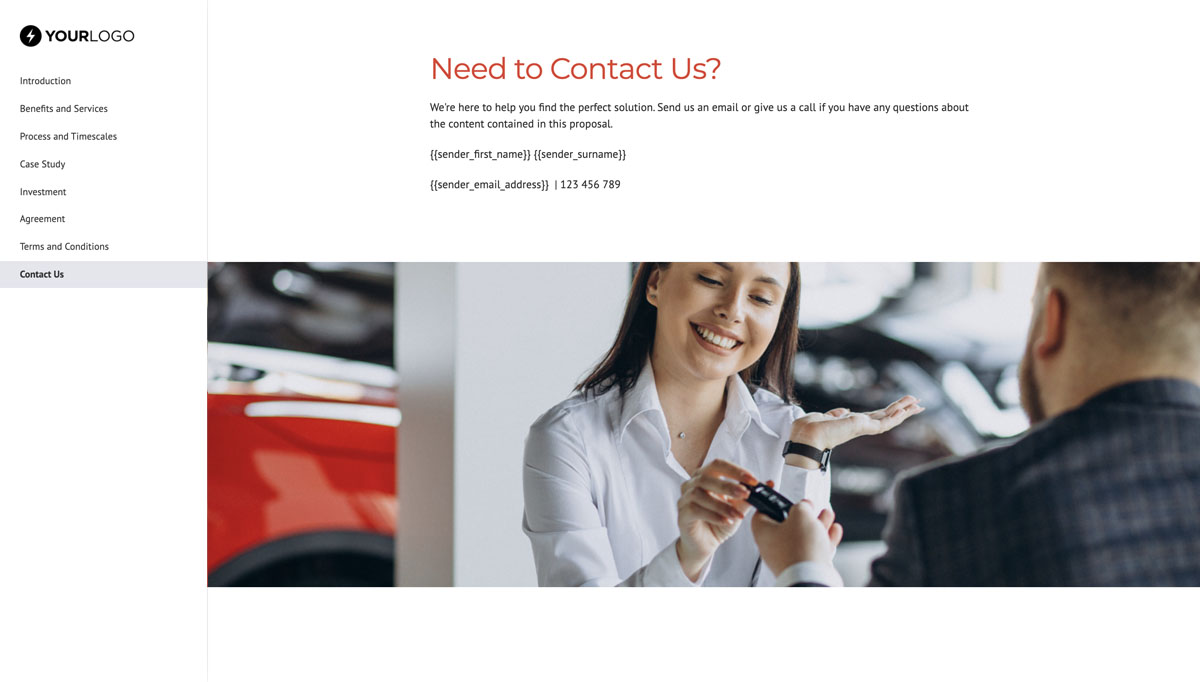The image showcases a website layout with a standard navigation bar on the left-hand side and its content on the right. The navigation bar has a white background and starts with "Your Logo" at the top. Below it, in sequential order, are the navigation links: "Introduction," "Benefits and Services," "Processing Timescales," "Case Study," "Investment," "Agreement," "Terms and Conditions," and "Contact Us" (highlighted in gray).

The main content on the right side features a large, bold text reading "Need to Contact Us?" in red, followed by, "We're here to help you find the perfect solution. Send us an email or give us a call if you have any questions about the content contained in this proposal." Below this message, there are placeholders for user input: "(sender_first_name)", "(sender_surname)", "(sender_email_address)", and a line indicating where the information should be filled in.

Additionally, there is a stock image of a woman with light skin and brown hair, wearing a white collared shirt, smiling while handing a card to a man. The setting appears to be a shop, and the woman exudes a friendly and professional demeanor.